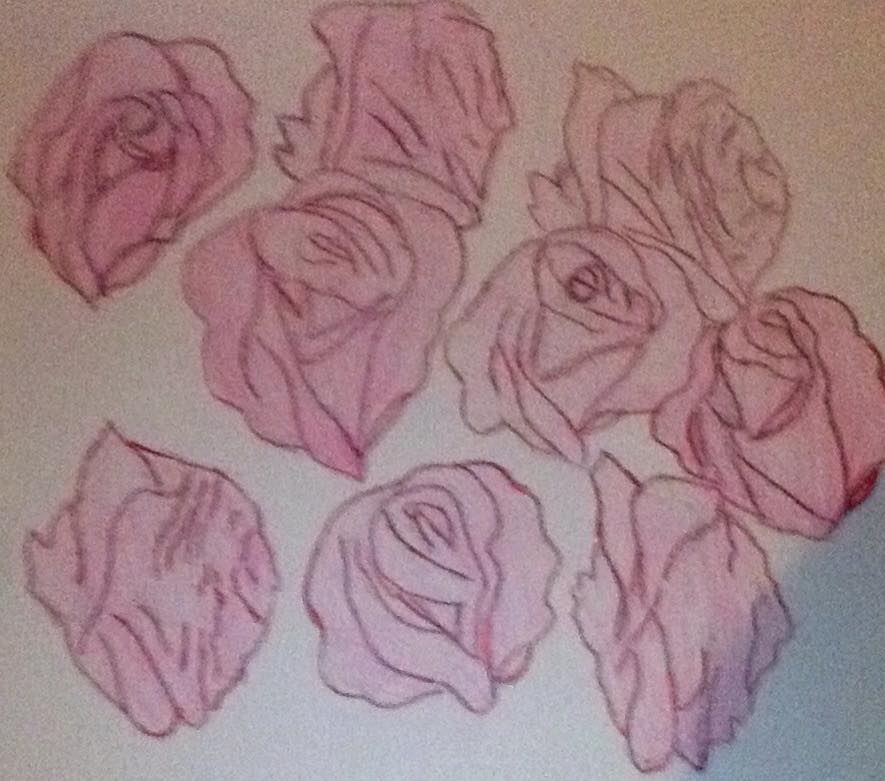This intricate square drawing on off-white paper features nine meticulously illustrated roses, each depicted solely as the bloom itself without stems or leaves. The roses, each outlined in black, showcase delicate, pink petals that offer a striking contrast against the background. These blossoms are thoughtfully arranged, each rose facing a unique direction to add dynamic movement and visual interest to the composition. Some roses are angled towards the top left, others towards the far right, while several are oriented fully upward. The varied positioning of the roses creates a captivating, almost dance-like pattern across the square canvas, highlighting the natural beauty and individuality of each bloom.